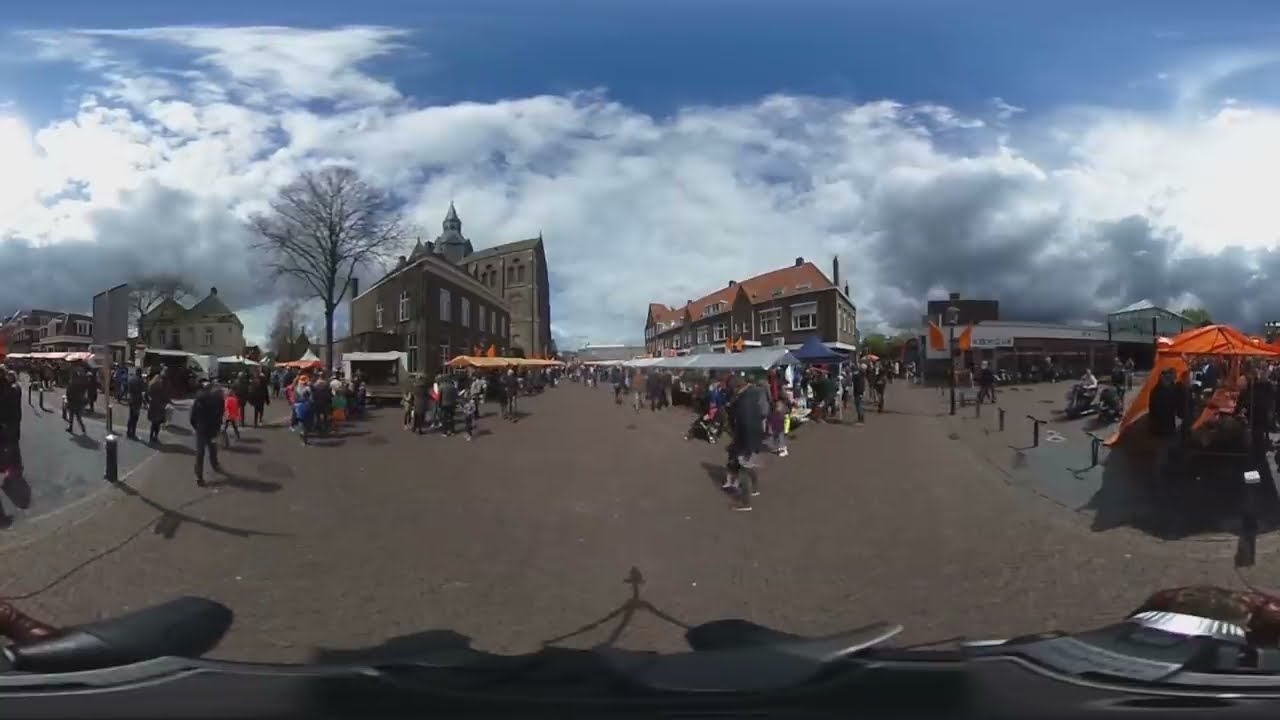This image is a detailed panoramic view of a bustling outdoor scene in a European-style town square, likely taken with a fisheye lens due to the curvature and wide-angle perspective. The setting appears to be a carnival or festival, with the central focus on a large, lively crowd of at least a hundred people milling about. The ground is a brick walkway, and numerous tents and umbrellas are set up, predominantly on the right side of the image.

Towards the upper part of the image, the sky is mostly covered in clouds, hinting at cool, late evening weather. The crowd includes individuals wearing coats, suggesting the temperature is on the cooler side. Among the crowd, there are notable elements such as people walking, some with strollers, and a couple holding hands. In the background, a series of two-story buildings, typical of German or Italian architecture, can be seen, one of which has a prominent spire or steeple on the center-left. A tree is also visible next to this building, adding a touch of greenery to the urban landscape.

On the bottom center of the image, the shadow of a tripod is noticeable, indicating that the photo might have been taken using a mounted camera. Concession tents with various roof colors—orange on the left and silver on the right—are set up throughout the background, indicating the presence of vendors and adding to the festive atmosphere. There is a specific orange-roofed concession tent prominently visible on the extreme right. The scene is lively and crowded, encapsulating the vibrancy of a town fair in what appears to be a small European town.